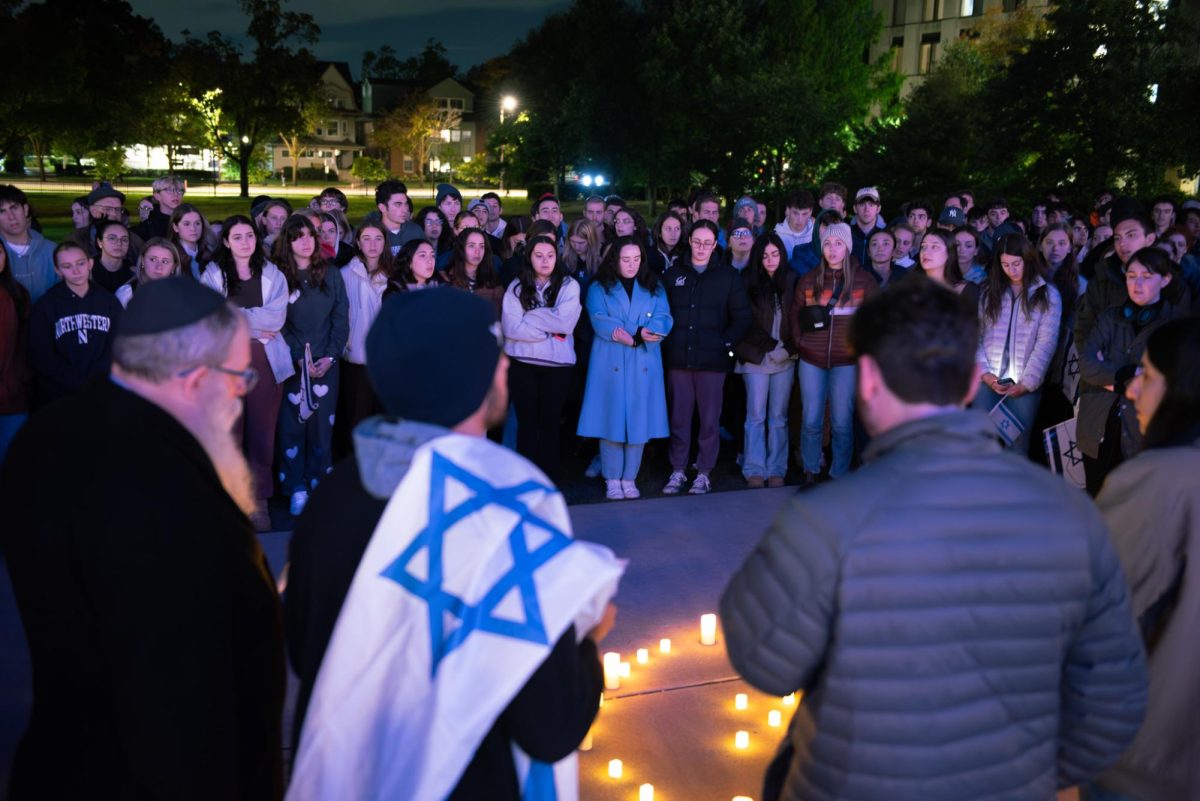This color photograph, taken at night, captures a somber candlelight memorial, possibly on a college campus. The scene is dimly lit except for the artificial lights illuminating the gathering. A crowd, predominantly young people dressed in large overcoats, long-sleeved sweatshirts, and jackets, forms a circle around the candles arranged in a pattern on the sidewalk. 

In the foreground, four individuals stand with their backs to us. One of them has an Israeli flag draped over his right shoulder, and beside him stands a man who appears to be a rabbi, distinguished by his long white beard, gray hair, and black skull cap. He wears a big black overcoat, adding to the solemnity of the event.

Beyond these central figures, more attendees can be seen, their faces clearly lit by the candlelight, all looking somberly down at the candles. In the background, various buildings, including large university-like structures and houses, frame the scene, contributing to the impression that this memorial is taking place on a campus. The atmosphere suggests a chilly night, evidenced by the warm clothing of the participants.